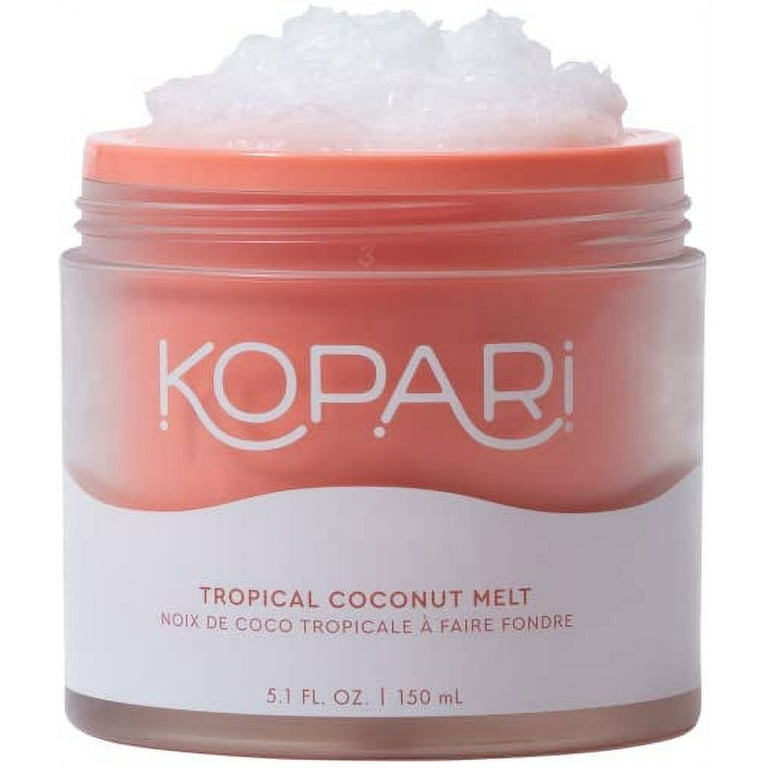The image portrays a beauty product pod positioned against a white background, reminiscent of a retail website. The canister, designed in portrait orientation, features an open mouth devoid of a lid, revealing an overflowing white, coconut cream substance. The upper section of the container is a light salmon pink, contrasted by a white wavy band that encircles the exterior. Displayed prominently on the band in swoopy letters is the brand "Kopari." Beneath the brand name, in smaller capitalized letters, it states "Tropical Coconut Melt" with the French translation "Noix de Coco Tropicale à Faire Fondre" directly underneath. The container, which has a capacity of 5.1 fluid ounces (150 milliliters), is detailed with a thin dark brown stripe running along the very bottom edge, adding to its visual appeal.